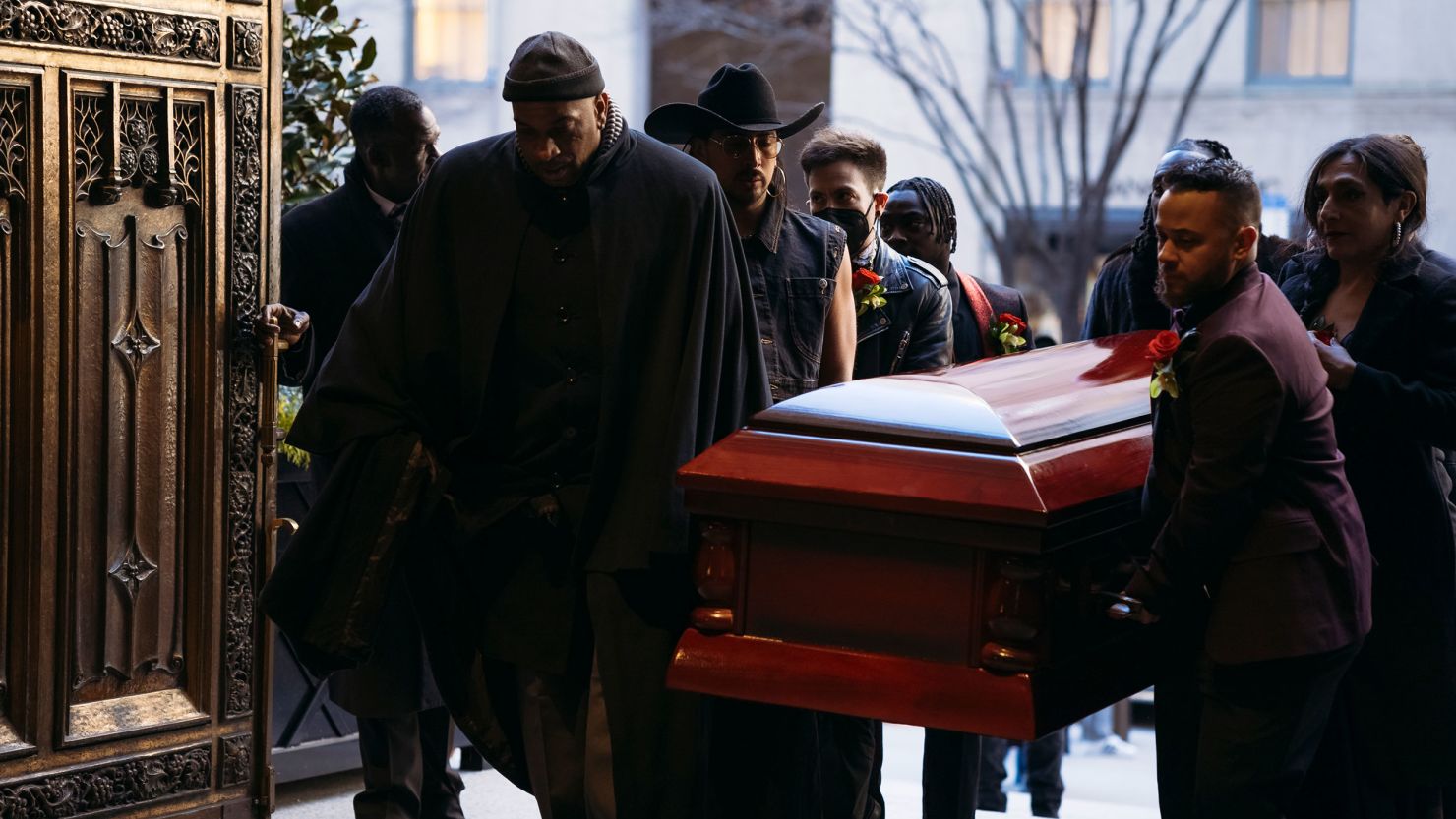In the high-quality, professional image of a funeral scene, a shiny mahogany wood casket is being carried by seven men and one woman, all dressed in darker colors. The group is moving through a set of ornate doors with gold designs, likely leading into a building, possibly a church. Among the pallbearers, the man at the front left is tall and wears a beanie, while the man directly behind him sports a black cowboy hat. Three men have roses in their handkerchief pockets. The background features onlookers, a white building with window borders, and a leafless tree, all slightly blurred to keep the focus on the somber procession.